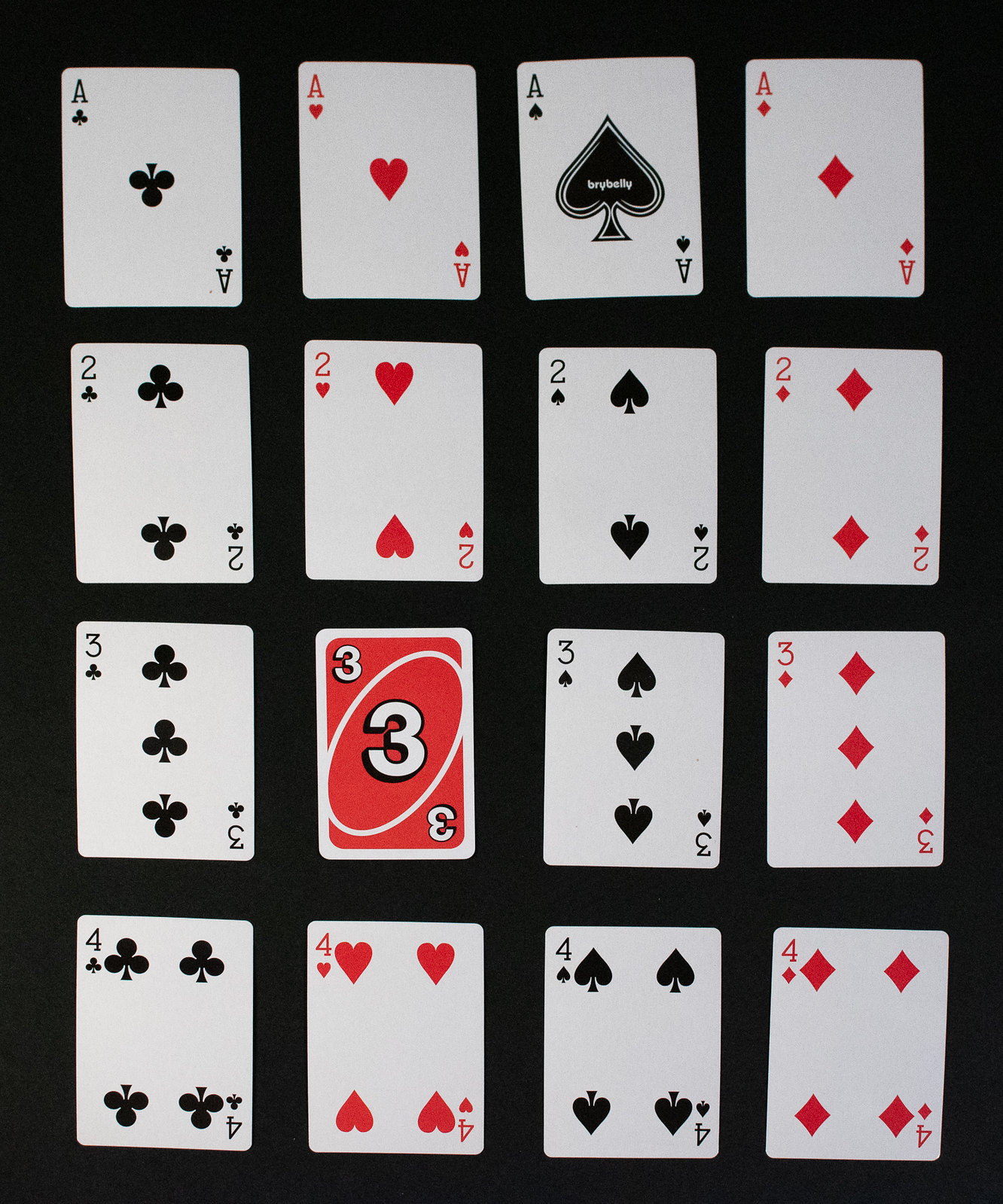The image features a neatly arranged 4x4 grid of playing cards set against a black background. Although the arrangement appears meticulous, it is not perfectly aligned, hinting at manual placement rather than digital generation. Each card has a white background with its respective suit and number prominently displayed. 

From left to right, top to bottom:
- The first row consists of an Ace of Clubs (black), Ace of Hearts (red), Ace of Spades (black), and Ace of Diamonds (red).
- The second row features a Two of Clubs (black), Two of Hearts (red), Two of Spades (black), and Two of Diamonds (red).
- The third row includes a Three of Clubs (black), an atypical card that deviates from the standard design—a red card labeled with a '3' at the top and bottom, and a large '3' encircled in the middle, followed by a Three of Spades (black) and a Three of Diamonds (red).
- The fourth and final row displays a Four of Clubs (black), Four of Hearts (red), Four of Spades (black), and Four of Diamonds (red). 

Overall, the cards are aligned in a structured grid, showcasing each suit and number up to four, with the exception of the single non-standard card in the third row.